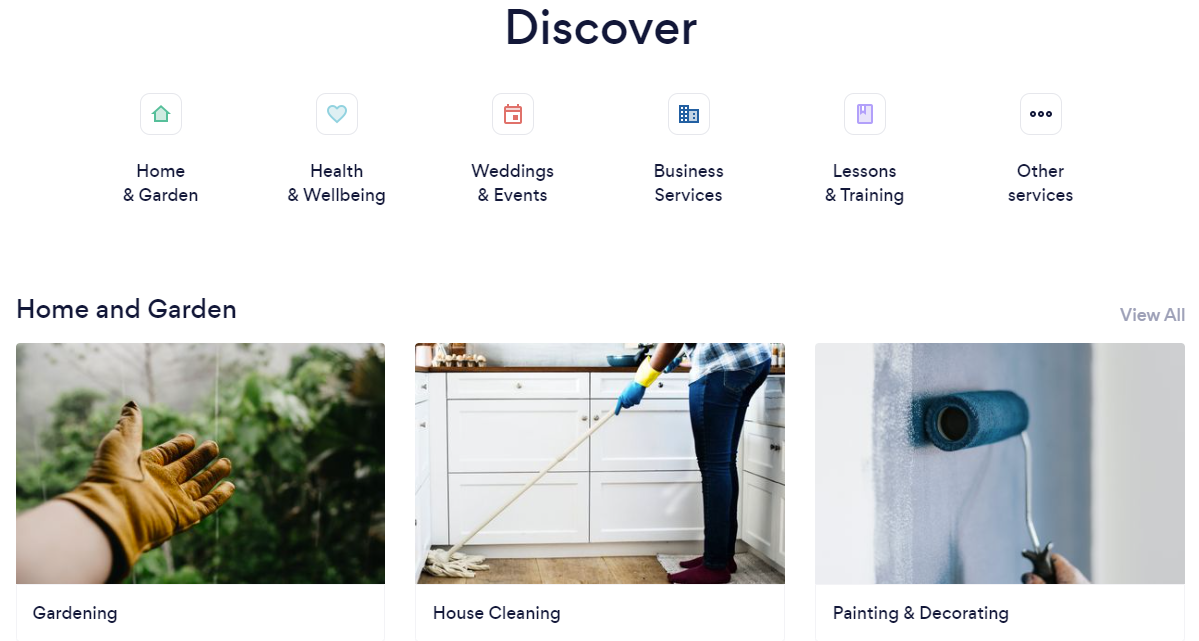The image is a screenshot featuring a webpage that prominently begins with the word "Discover" in black text centered at the top. Immediately below this header, there is a horizontal menu showcasing various categories, each represented by an icon. The categories listed are: 

1. **Home and Garden**: Depicted with a home icon.
2. **Health and Wellbeing**: Represented by a heart icon.
3. **Wedding and Events**: Illustrated by a calendar icon.
4. **Business Services**: Denoted with a building icon.
5. **Lessons and Training**: Shown with a notebook icon.
6. **Other Services**: Characterized by an icon of three horizontal dots.

Each category has further submenus under it. The category "Home and Garden" is highlighted, revealing three sub-sections presented horizontally below it:

1. **Gardening**
2. **House Cleaning**
3. **Painting and Decorating**

Each subsection is contained within a distinct box, indicating that these are specific services available under the "Home and Garden" category.